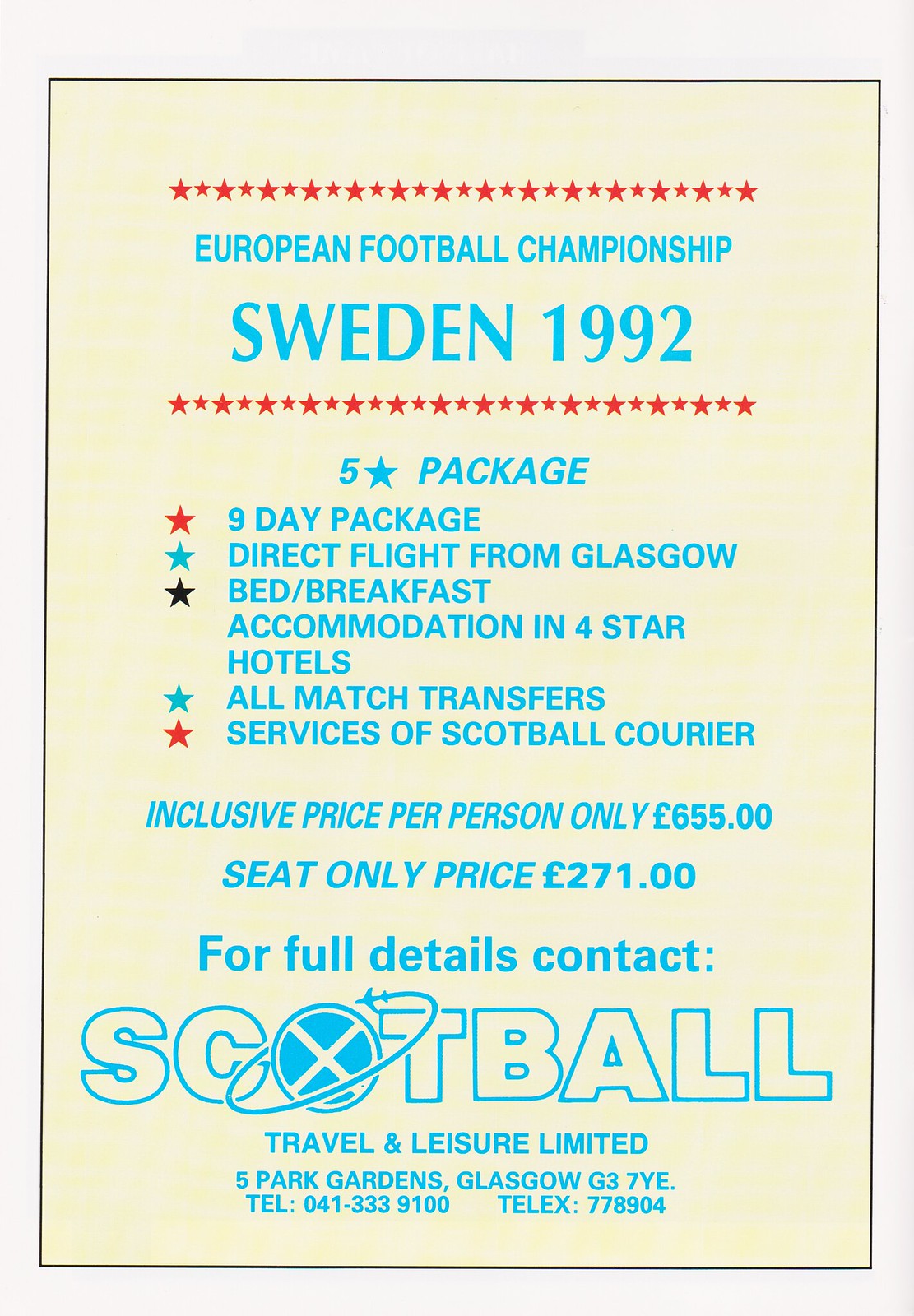The advertisement features a beige background bordered by red stars and presents in striking blue text: "European Football Championship Sweden 1992." The enticing offer, labeled as a five-star package, details a nine-day itinerary that includes a direct flight from Glasgow, bed and breakfast accommodation in four-star hotels, all-match transfers, and the dedicated services of Scott Ball Courier. It provides an inclusive price of £655 per person or a seat-only price of £271. The advertisement prominently displays the Scott Ball Travel and Leisure Ltd. logo, with a plane circling the 'O' in 'Scott Ball'. For full details, the contact information is provided as: Scott Ball Travel and Leisure Ltd., Five Park Gardens, Glasgow, G3 7YE, Tel: 041-333-9100, Telex: 77890.